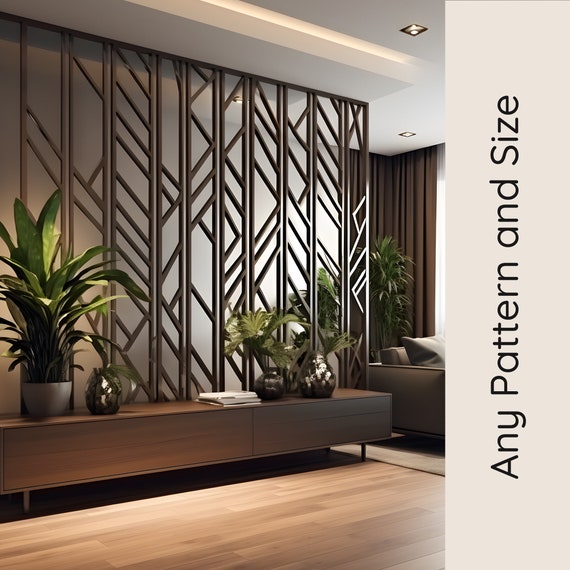This vertical color photograph captures the interior of a luxurious commercial space, possibly a hotel lobby or a high-end office waiting room. The two-story space has a sophisticated, brown-and-white color scheme. Dominating the scene is an elongated, Scandinavian-style table, which appears like three coffee tables joined together. This table is adorned with lush, expensive-looking tropical plants in an assortment of white, silvery, and dark brown pots. Strewn across the table are several professional photography books, adding a cultured touch.

The room features tall, artistic wooden pillars and a hardwood floor with a light stain, complemented by a beige rug. Near the right edge of the image, a partial view of a large brown leather chair or sofa is visible. The setting is highlighted by high ceilings and large curtains on the right-hand side, which add to the grandiosity of the space. A stained dark wooden trellis in the background and a beige banner that vertically displays text further enhance the room's elegant decor.